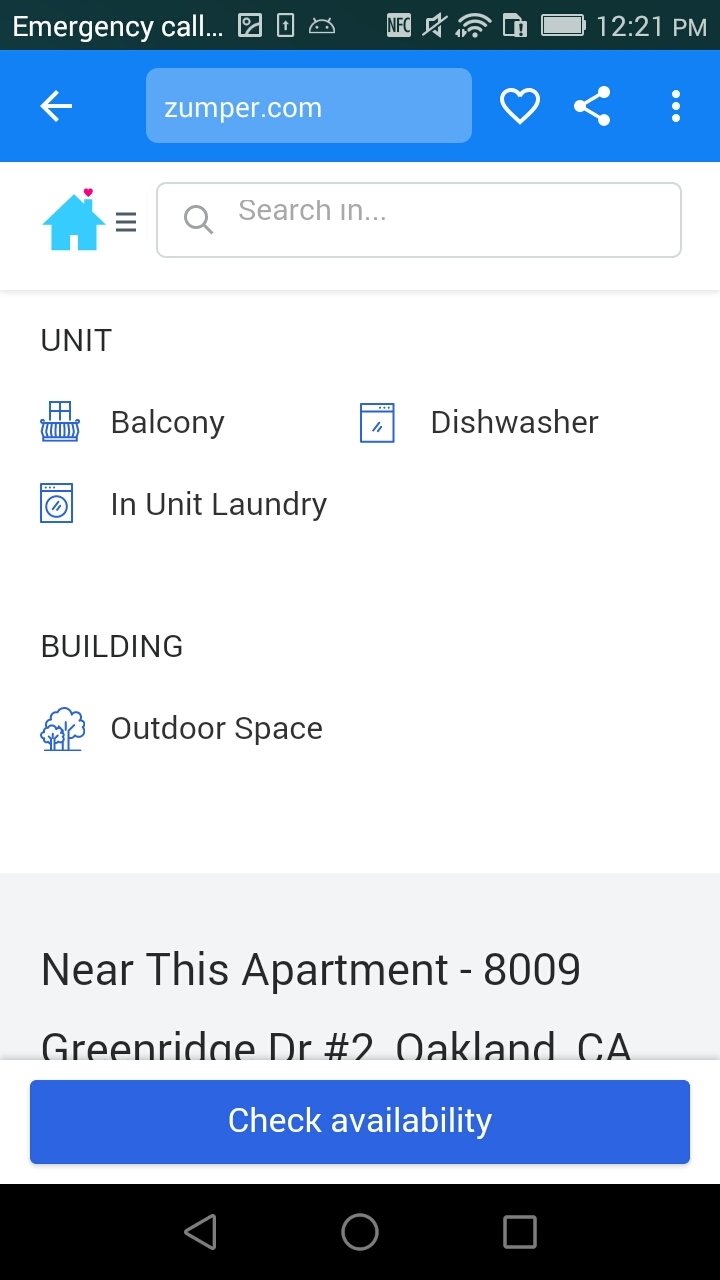The image appears to be a screenshot from an Android phone, identifiable by the navigation bar at the bottom, which features a left-pointing arrow, a circular home button, and a square multitasking button. At the top, the status bar displays "Emergency call" alongside various icons: NFC, silent mode, Wi-Fi, SD card, and a fully charged battery, with the time reading 12:21 PM.

Immediately below the status bar, there's a blue strip featuring a left-pointing arrow and a search box containing the URL "zumper.com". To the right of the search box are three icons: a heart (likely for bookmarking the page), a share button, and a three-dot menu for additional settings.

The main content area transitions to a white background, starting with an icon of a small house with a red dot above its chimney beside a hamburger menu symbol (three horizontal lines) and a blank search box. Beneath this, there is a section labeled "Unit" that lists various amenities through small icons:
- Balcony, represented by a balcony with a window.
- In-unit laundry, depicted by a washing machine.
- Dishwasher, shown with a dishwasher icon.

Following this, a section labeled "Building" shows an icon of trees with the text "Outdoor space."

A prominent gray box contains detailed text: "Near this appointment - 8009 Green Ridge Drive, #2, Oakland, California."

Finally, a large blue button at the bottom of the screenshot reads "Check availability."